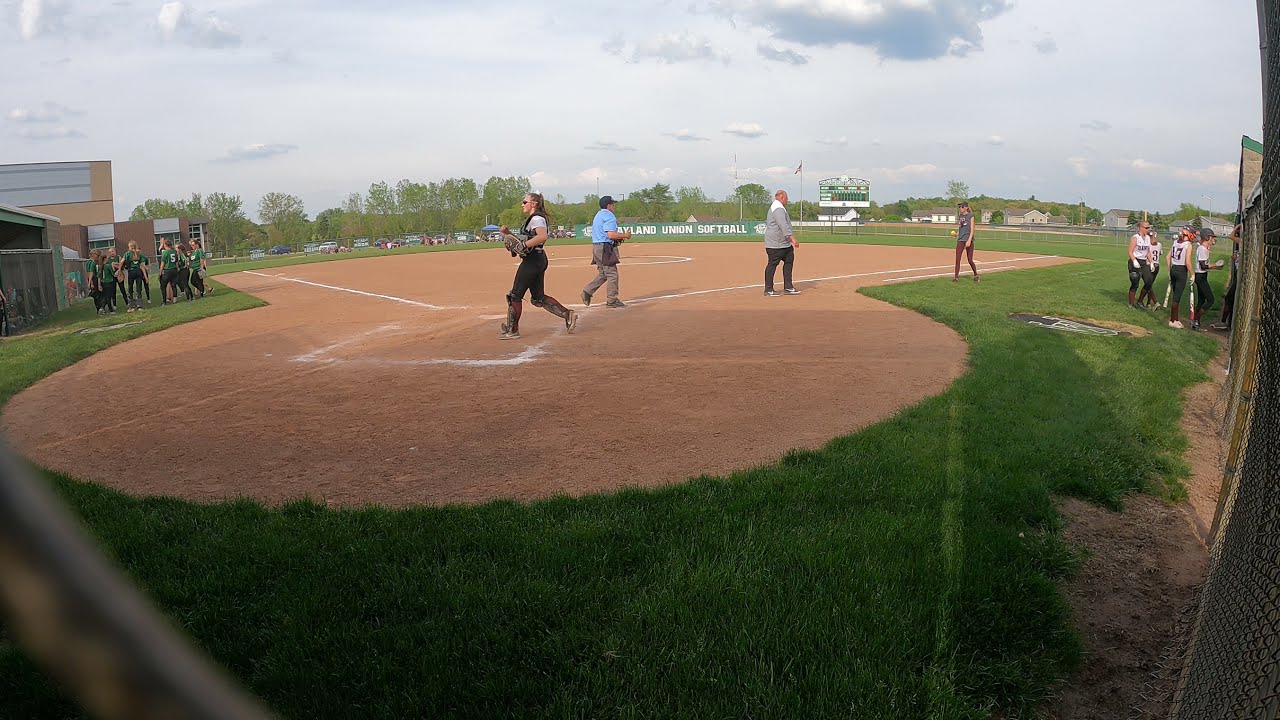The image captures the scene of a softball game, potentially part of a league, with two teams preparing for or winding down a match. The field is well-kept, with green grass stretching across the playing area. Off to the left, a team of girls in green shirts and black pants stands together, while on the right, members of another team donning white or gray shirts and black pants are gathered. Visible numbers on the shirts include 3 and 17.

In the center of the field, a girl wearing black overalls over a gray shirt and sunglasses is running towards the left, presumably towards a base or to the dugout. Nearby, two men can be seen: one in a blue shirt and gray pants with a sack around his waist walking towards another man in a gray shirt and black pants. Additionally, a girl holding a white cup walks beside the field.

An umpire and what appears to be a coach are positioned centrally, engaged in conversation or decision-making. In the far background, partially obscured by the umpire, a sign reads "Union Softball," with the first word potentially being "Maryland" but not entirely clear. The image conveys the lively and organized atmosphere of a competitive softball event, with players, coaches, and official personnel all contributing to the unfolding scene.